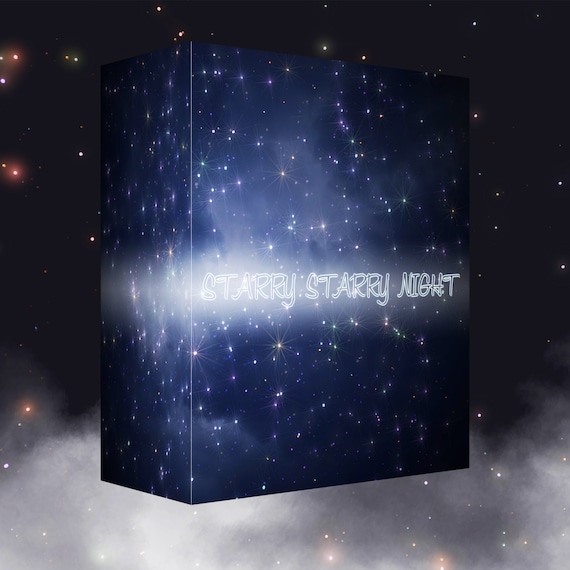The image depicts an illuminated, vertically oriented game box titled "Starry Starry Night" in prominently framed white lettering resembling hollow bubble letters. The box’s design is predominantly blue and black, adorned with a luminescent sky full of stars, giving a sense of a crystal-clear night devoid of light pollution. A distinct light reflection is seen on the left side of the title, adding to the box's bright and shiny appearance. The lower part of the box features a nebulous or cloudy area in the cosmos where stars are visible through the cosmic dust and fog, creating a textured backdrop. The box appears to float against a similarly star-strewn, cosmic background that transitions from a darker, dimmer sky with cloud cover to a more vibrant, star-packed region higher up. Some stars in the image appear red and yellow, contributing to the vivid and deep space atmosphere. The overall presentation, with its cosmic elements and detailed starry themes, suggests that the box is likely showcasing a product, possibly a board game.